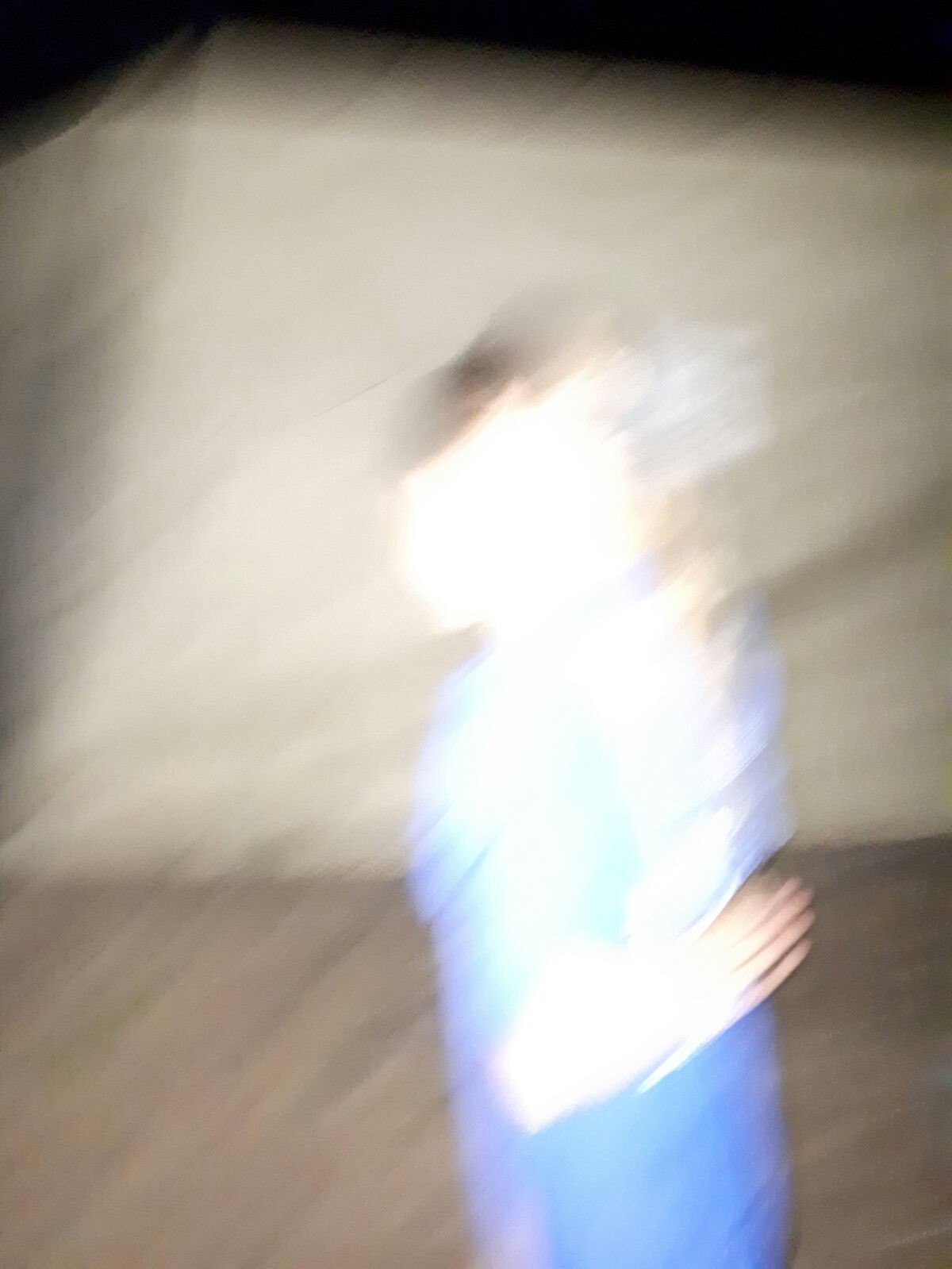This vertical, portrait-oriented photograph is extremely blurry, likely due to camera movement during capture. The image features a significant section of white light that covers almost three-quarters of the photograph, making it difficult to precisely discern the subject. The blurred figure at the center appears to be a person, potentially facing to the right, with the outline of their head and a portion of their right hand visible. The person seems to be wearing a blue shirt, as indicated by the light blue sections at the bottom and throughout the image. Above these blue areas, the heavy blur distorts the figure, blending into the white flash. The background contains a darker white base and a lighter white region with lines suggesting either a building or a tent structure. The overall effect is compounded by streaks of light that run from left to right and up to down across the image, enhancing the obscurity and adding to the chaotic composition.